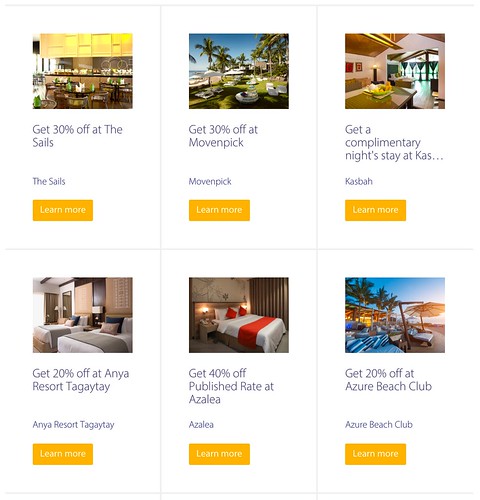Here is a cleaned-up and detailed caption for the described image:

---

The image consists of six promotional pictures arranged in a 3x2 grid. Each picture features an offer and a corresponding "Learn More" button in orange with white text.

- **Top Left:** An offer for "Get 30% off" with the background showing the cozy interior of a stylish restaurant.
- **Top Center:** An offer for "Get 30% off at Movenpick," showcasing a serene outdoor setting with verdant green trees, a blue ocean, lush grass, and a few scattered white chairs.
- **Top Right:** An offer for "Get a complimentary night stay at Casbah," depicting a tastefully decorated room with white walls and elegant black curtains.
- **Bottom Left:** An offer for "Get 20% off at Anya Resort Tagaytay," featuring a tranquil room with two neatly made beds adorned with white beddings and gray blankets.
- **Bottom Center:** An offer for "Get 40% off published rates at Alera," highlighting a chic room with a bed dressed in white linens and accented with red pillows.
- **Bottom Right:** An offer for "Get 20% off at Azura Beach Club," showing a picturesque coastal scene with green trees and blue boats near the ocean.

Each image captures the unique ambiance of its respective location, enticing viewers to explore these offers.